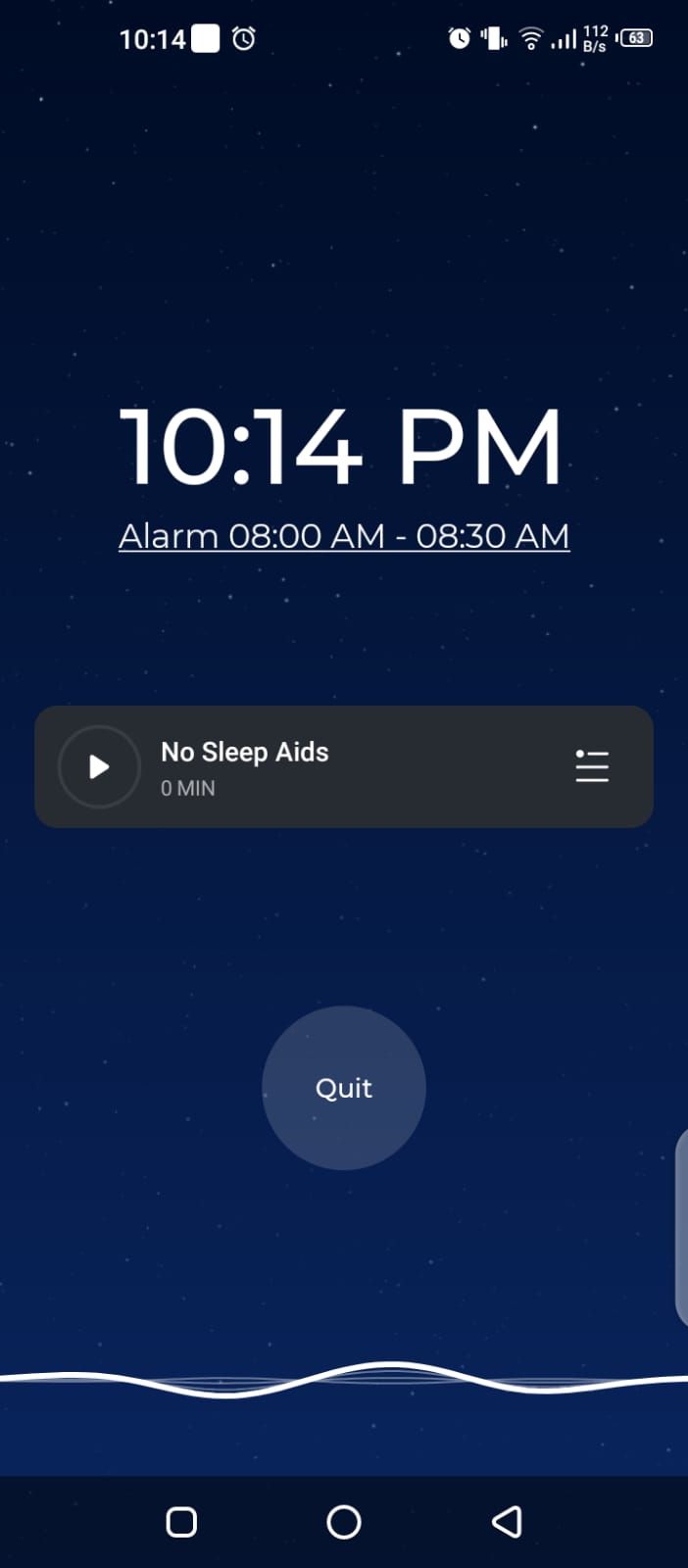This image is a screenshot from a smartphone or tablet, featuring a dark blue background. At the top, it displays "1014" in white text inside a square, accompanied by a clock icon. On the right-hand side, there appears to be multiple notifications; one indicating an active clock setting, and another showing that vibration mode is on, represented by a rectangle with lines at the top left and bottom right corners. The wireless signal strength shows three out of four bars, indicating a strong connection. The cellular signal strength is full, labeled as "112BSS" in bits per second (with a capital "B"), and the battery icon, pointing left, reads 63%, showing the remaining battery life.

Centrally positioned in bold white text is "10:14 PM" with an "Alarm 8:00 AM to 8:30 AM" text below it, underlined by a line. There is also a black rectangle pop-up with a faded gray circle containing a white arrow pointing to the right. Bold white text within the pop-up states "No sleep aids," and beneath this in gray, it says "0 minutes." To the right of the pop-up, there is a white circle with three lines and another semi-transparent white circle below it, with "Quit" in bold white text. Below this is a line accompanied by smaller white lines and at the bottom, icons for a square, circle, and left-pointing triangle rest above a black bezel.